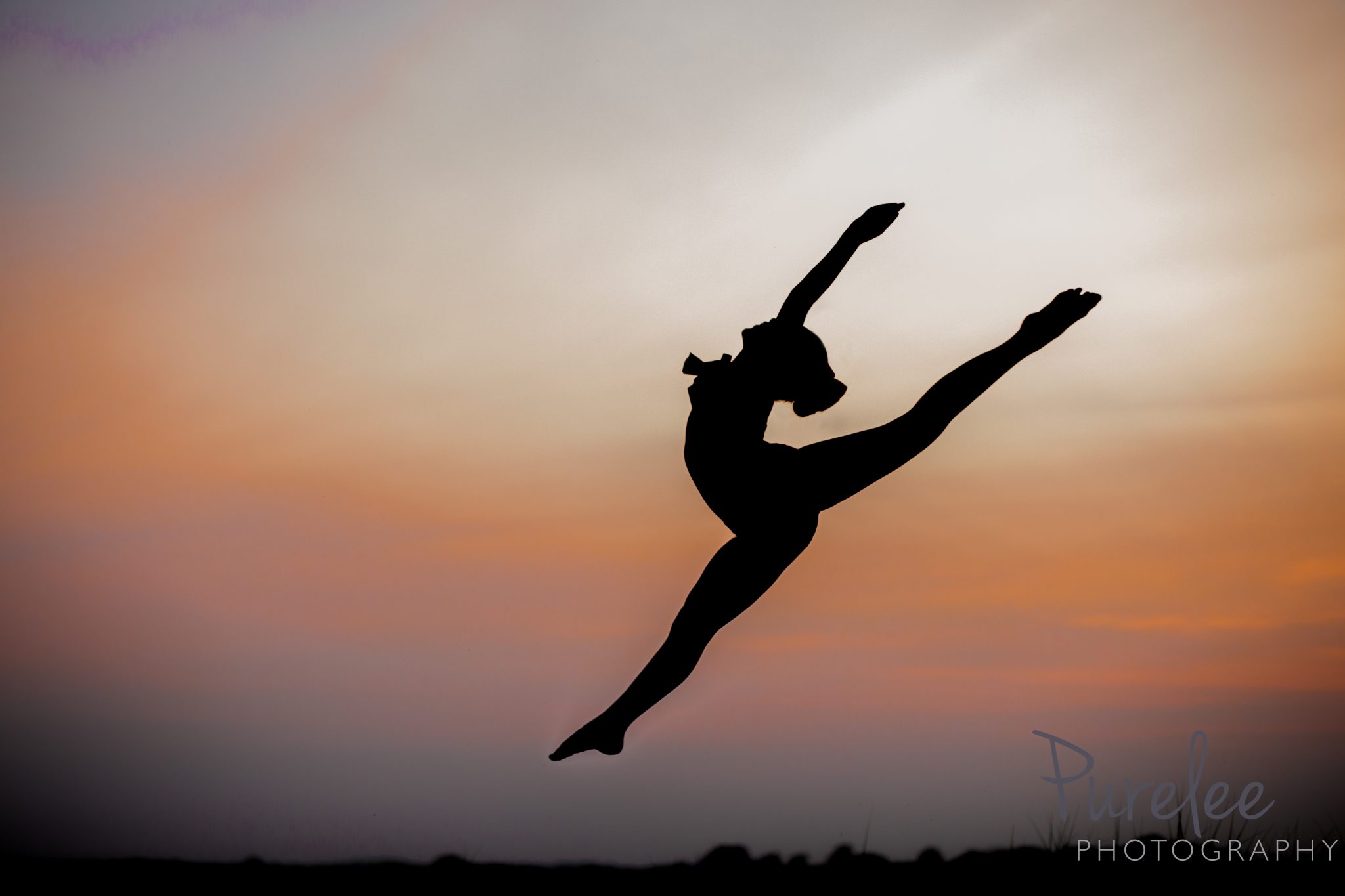In this stunning photograph, the silhouette of a female dancer or gymnast is captured mid-leap, seemingly suspended in the sky. She is performing an arabesque with an extreme backbend, her left leg lifted high and parallel to her arched back, and her pointed toes accentuating the graceful pose. Her right arm is extended upwards, creating a fluid line from her fingertips to her toes. The silhouette is crisply defined against the vibrant hues of an evening sky, which transitions from the muted grays and pinks near the horizon to rich oranges and violets above. The lower portion of the image features a contrasting black background, highlighting the striking silhouette. On the bottom right corner, the logo "PUREE Photography" is elegantly displayed in white cursive lettering, adding a professional touch to this breathtaking moment.